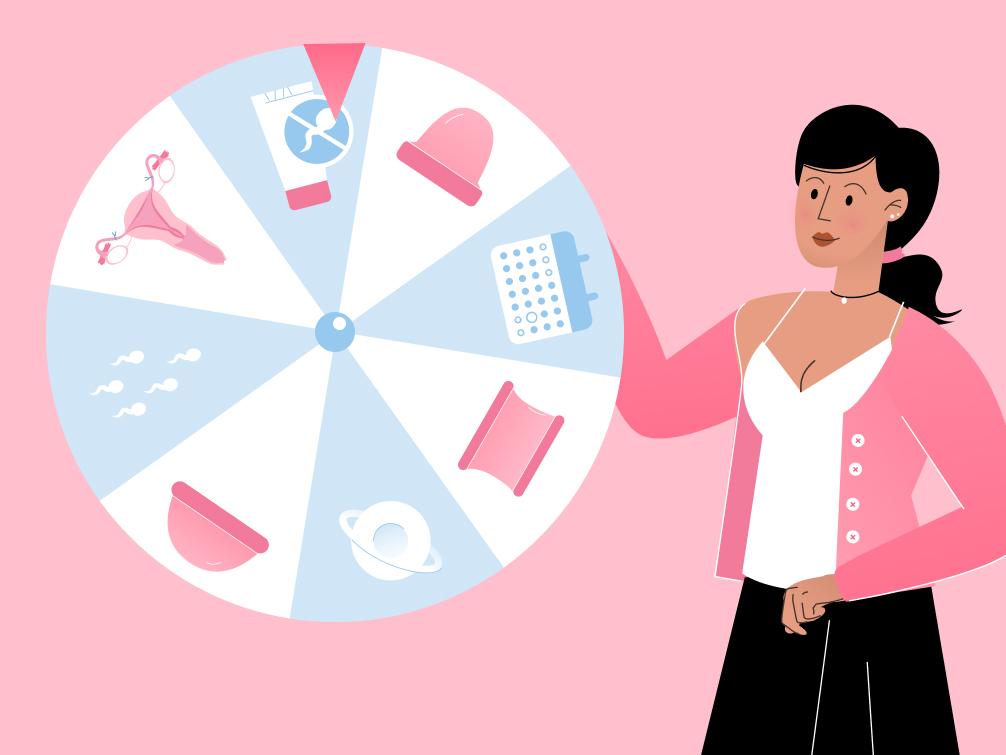The image is a detailed digital drawing with a light pink background, measuring approximately six inches wide by four to five inches high. Dominating the right side of the picture, a cartoon woman stands from the knees up. She has dark hair tied back in a ponytail with a pink band, light skin, and is dressed in a pink long-sleeve sweater with white buttons over a white halter top, paired with a black skirt. She looks to the left, her right hand extended and bent at the elbow, reaching behind a large circle positioned on the left side of the image. 

The large circle resembles a roulette wheel, sectioned into eight wedges with alternating white and light blue backgrounds, each depicting symbols related to contraception. At the top of the wheel, there is a white tube with a red cap, followed clockwise by a blue circle containing a sperm with a white line through it, indicating spermicide. Next is a depiction of a pink cup and at the three o'clock position, a pack of birth control pills. Continuing around, there is another pink tube at the five o'clock position, a white circle with a band around it at six o'clock, a different style of pink cap at seven o'clock, white sperms at nine o'clock, and finally, a pink uterus image between ten and eleven o'clock. At the top of the wheel is a triangular dial pointing downwards, suggesting the wheel can be spun.